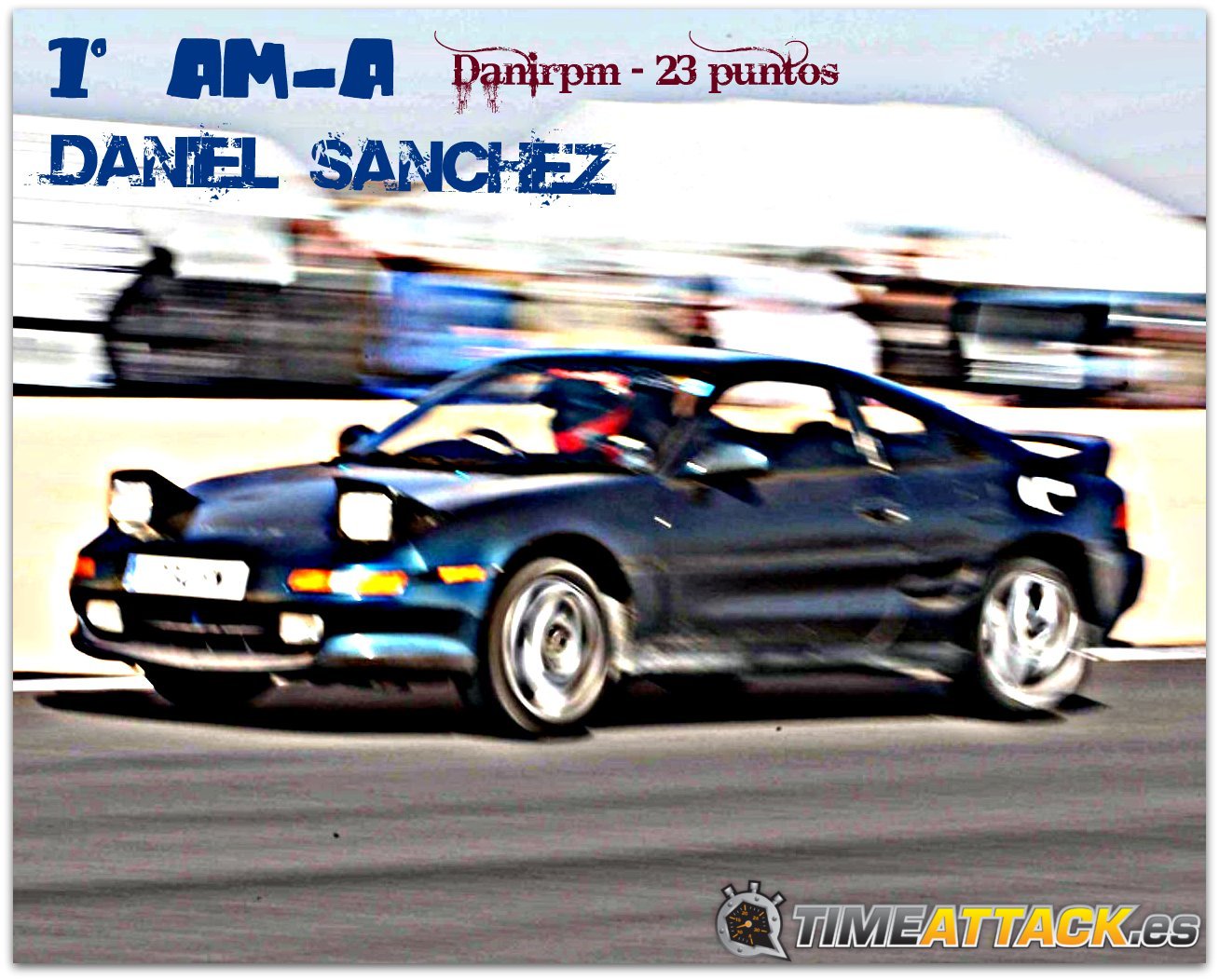The image showcases a sleek, dark blue sporty passenger car speeding along a track, its raised headlights beaming brightly. The rapid motion of the vehicle is emphasized by the blurred yellow wall in the background, creating a dynamic sense of speed. At the top left of the image, bold blue letters spell out "1M-A" and just below that, "Daniel Sanchez" is also in blue. To the right of the name, in striking red letters, it reads "Danner PM - 23 Puntos." In the bottom right corner, a silver stopwatch icon is displayed alongside text that reads "Time Attack .ES" in a mix of silver and blue. The car appears to be moving very fast, and the overall graphic style has an animated, almost pop-art feel. The background primarily focuses on the car, with no visible driver, and minimalistic, abstract details.